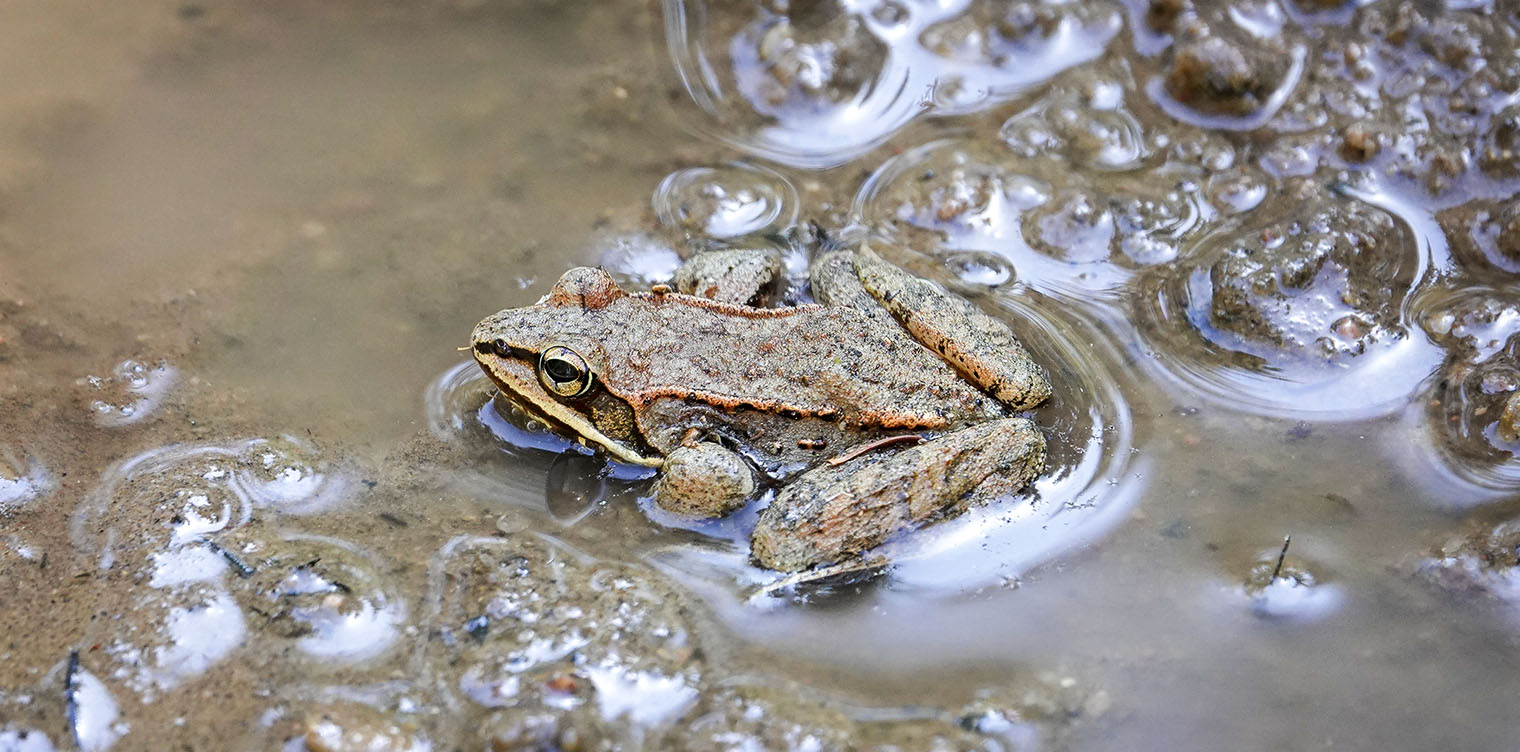The photograph captures a close-up view of a large brown frog with yellow and gray spots, crouching low in a small, shallow puddle filled with mud and gravel. The frog, facing towards the left, displays two distinctive orange-colored ridges along its sides, while its two long hind legs are bent and pressed up against its body. The frog's underbelly, including its stomach and chest, is a whitish-yellow hue. Its striking yellow and black eyes add to its alert demeanor as it appears on the verge of a leap. The murky water, indicative of a swamp-like environment, showcases water bubbles and soil beneath, reflecting the daylight that illuminates the scene. The photograph, taken from an angled perspective, primarily reveals the left and top sides of the frog, highlighting its intricate details against the muddy backdrop.